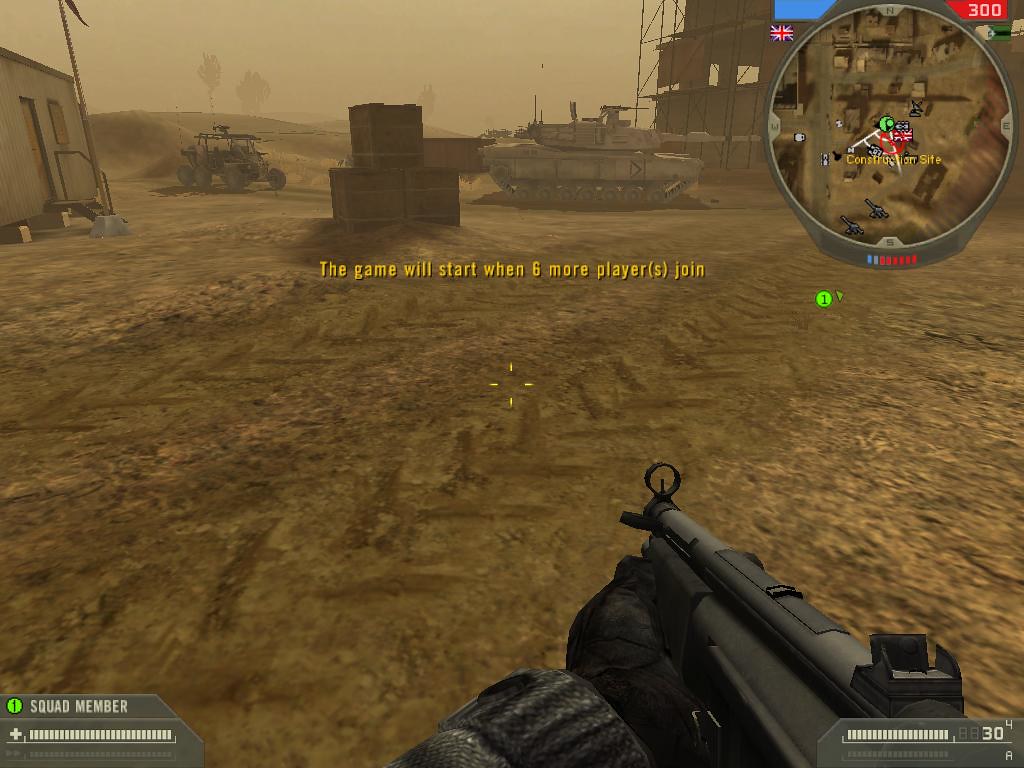The image appears to be a screen capture from a first-person shooter video game set in a military environment. The scene is a desert landscape featuring a tank in the distance and a military ATV to its left. Surrounding the vehicles are several structures, likely warehouses or industrial buildings, positioned on both sides of the tank. In the foreground, the perspective suggests the playable character, evident by the visible gloved hand gripping the muzzle of a firearm. Additionally, a "Squad Member" label is visible in the lower left corner, indicating team-based gameplay elements.